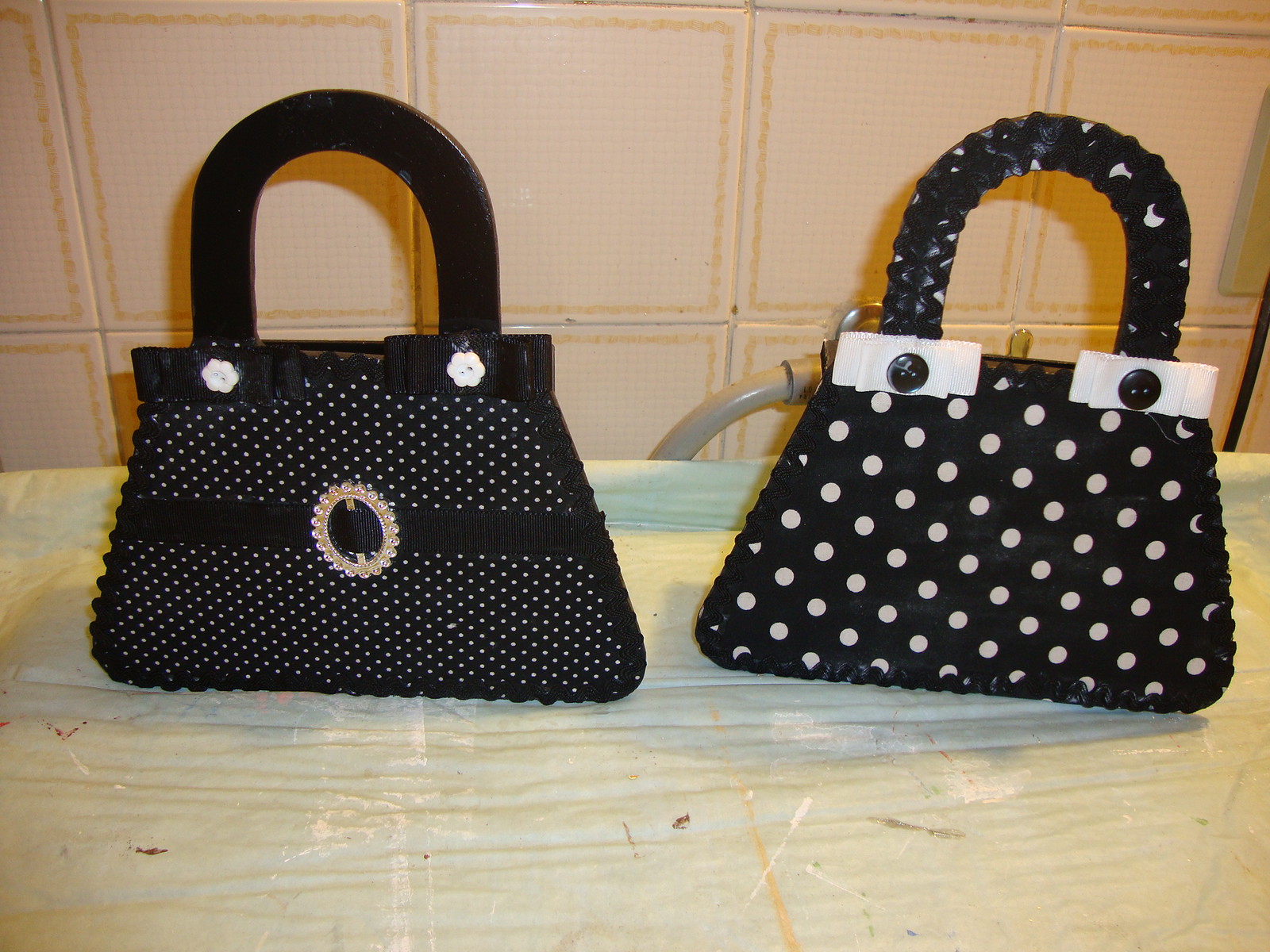This is a color photograph capturing a wooden tabletop set against a tiled wall, with two black purses prominently displayed in the foreground. The background reveals a wall adorned with 12-inch by 12-inch tiles in shades of beige, light pink, light orange, light tan, and light cream, detailed with grey grout and a subtle orange trim. The tabletop, made of light-colored wood, exhibits signs of heavy use, including numerous dents, scratches, and discolorations.

Both purses share a similar angular design, reminiscent of a truncated triangle. The purse on the left features a smooth black handle adorned with two white flower-shaped buttons centered in black bows. Its black body is patterned with small white polka dots, and it boasts a horizontal black ribbon embellished with an oval brooch circled by what appear to be rhinestones.

The purse on the right mirrors the same shape but includes a textured black handle decorated with white bows that have black centers. This purse has large white polka dots on its black body, contributing to the striking visual symmetry between the two accessories.